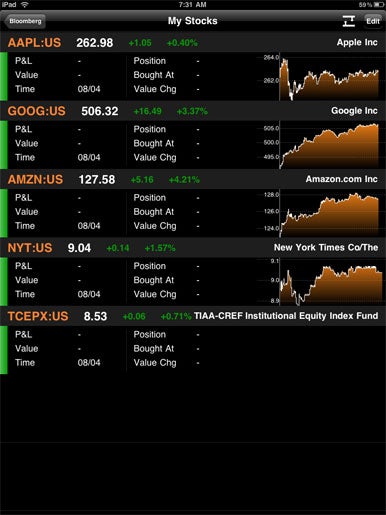The image is a detailed screenshot of a stock market tracking application captured on an iPad. The background is entirely black, enhancing the visibility of the details. At the top-left corner, the iPad status bar is visible featuring the Wi-Fi icon, while the battery level indicator is situated at the top-right, and the current time reads 7:31 AM.

Below the status bar, the interface of what appears to be the Bloomberg app is displayed. At the very top-center of the screen, the title "My Stocks" is prominently shown, indicating a personalized stock watchlist.

The main section of the image showcases a list of various U.S. companies, including Apple, Google, Amazon, The New York Times, and TCEPX. Each company's name is displayed in white text, followed by essential financial data. This includes their current stock prices, the direction of their movement (up or down), and miniature graphs representing the performance trends over a selected period.

Additional information such as the specific positions, their purchase prices, and overall worth of the stocks are meticulously arranged beneath each company's name, providing a comprehensive snapshot of their market standing.

Overall, the clarity and layout of the information, combined with the dark mode interface, make detailed stock analysis easily accessible.